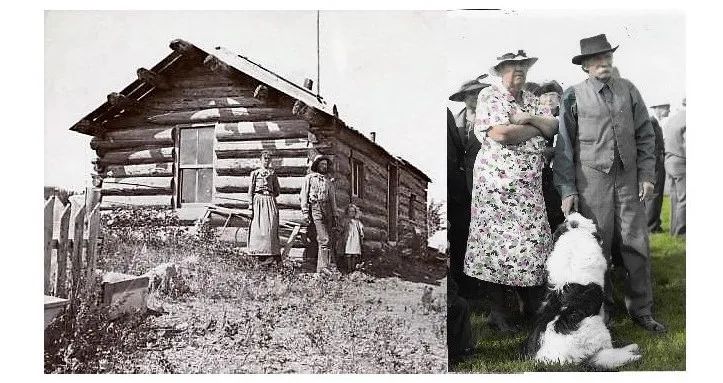This image is split into two distinct vintage photos side by side. The left photo, in black and white, depicts a rustic log cabin set in a prairie-like setting, illuminated by daylight. Prominently featured are a man in a hat, a woman in a long-sleeved dress, and a little girl standing at the corner of the cabin. Visible details include a window on the side, two additional windows, and a door at the front, with some dirt and grass surrounding the scene, and a small picket fence to the left of the house. A tall pole protrudes from the cabin’s roof, adding an intriguing element to the otherwise quaint setting.

On the right side, the color photo captures a sharply dressed elderly couple, the woman adorned in a floral dress and a hat, with her arms crossed, while the man wears gray slacks, a matching shirt, vest, and a dark hat. At their feet sits a black and white dog, its back facing the camera. The couple stands on a grassy area, with indistinct figures in darker grayscale tones visible in the background, creating a stark contrast and suggesting the photo may have had color added or been digitally remastered.